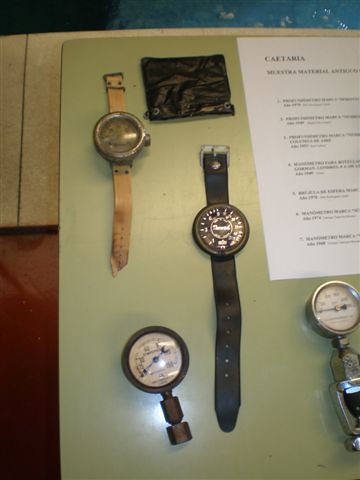The image depicts a collection of items placed on a green surface, possibly a table or desk. At the top of the surface lies a small black pouch, laying flat, which appears to be a wallet or carrying case. 

Adjacent to the black pouch on the left side is an antique-looking wristwatch. The watch features a cream-colored strap that appears very worn and a silver bezel that shows significant aging and tarnish. The watch face is obscured by a dirty and darkened glass covering, making it difficult to see any details.

Below the antique wristwatch and slightly to the right is another wristwatch. This one has a modern design with a black strap, black bezel, and black dial. The numbers on its face are white, but they are out of focus and unreadable.

At the bottom left of the arrangement is a metallic dial, likely a pressure gauge. It features a metal bezel and has a screw attachment at the bottom. The gauge has a white face with blue and red lettering, although the specifics of the text are indistinct.

Additionally, there is a piece of paper on the left side of the surface. The paper is white with black lettering, but the text is too small and out of focus to be legible.